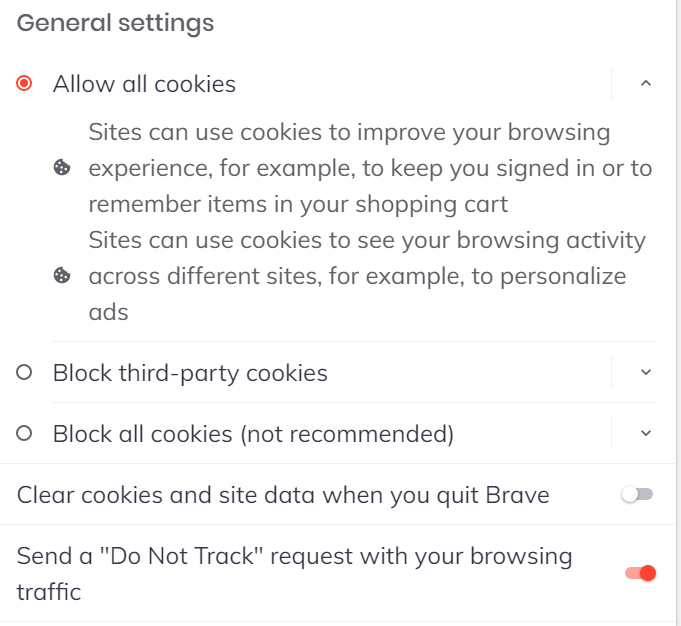The image displays a general settings menu on a web browser with a clean, white background and gray lettering. At the top, the heading "General Settings" is prominently displayed. Below this, a button labeled "Allow all cookies" is activated, highlighted in red. The accompanying description explains that allowing cookies can enhance the browsing experience by keeping users signed in and remembering items in a shopping cart. It also notes that cookies can track browsing activity across different sites for personalized advertising.

Additionally, several other options are listed:
1. "Block third-party cookies" – present but not activated.
2. "Block all cookies" – marked as not recommended.
3. "Clear cookies and site data when you quit Brave" – not activated.
4. "Send a 'Do Not Track' request with your browsing traffic" – this option is enabled, indicated by the button being red.

Each setting has a toggle button that switches from red (enabled) to white (disabled). A small icon of a bitten cookie symbolizes cookie-related settings, reinforcing the theme visually. The page has a straightforward and user-friendly layout, allowing users to easily manage their preferences for cookies and privacy.